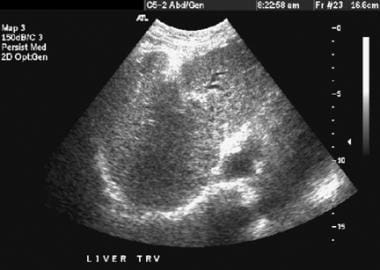This is a detailed black and white ultrasound image, displayed within a cone-shaped frame. A vertical scale with numbers ranging from 0 to 15 lines the right side of the image. The top left corner features several labels including "MAP3" and "150 BC3 persist med 2D op gen," accompanied by a timestamp reading "6:22 AM." Near the bottom left, the text "liver TRV" is clearly visible, indicating the specific area being scanned. The central portion of the ultrasound shows the familiar grainy, x-ray-like pattern typical of such scans, though the exact structures are not distinctly identifiable. The measurements in the image also include "16.6 cm" and "C5-2 abdomen gen." Overall, it appears to be a general abdominal ultrasound scan rather than one specifically of a baby.